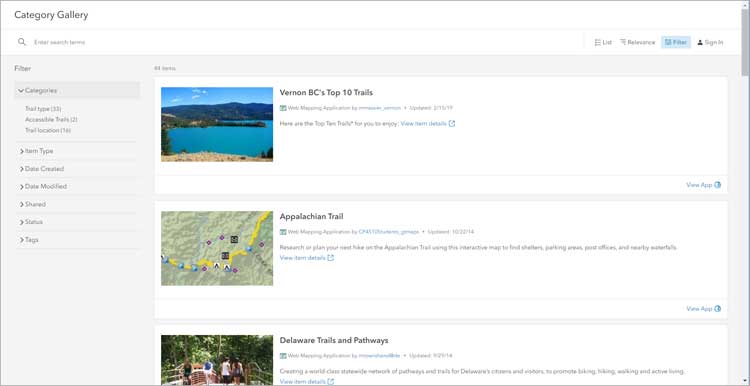The image appears to be a screenshot from a digital platform, possibly a photo application or a travel website, featuring a navigational interface on the left and a gallery of images showcasing trail recommendations. The navigation panel includes filters for 'Categories', 'Type', 'Date', and 'Shared.' 

At the top, under the 'Category' label, three highlighted images are displayed, each representing a different trail destination. The highlighted trails are "Vernon's BC Top 10 Trails," "Appalachian Trail," and "Delaware Trails and Pathways." The interface suggests that these are top recommended trails available for exploration.

The "Delaware Trails and Pathways" option appears to be particularly noted for its accessibility, potentially offering user-friendly or family-friendly hiking experiences suitable for beginners or those seeking less strenuous activities. However, further details about "Vernon's BC Top 10 Trails" are not provided, leaving its level of difficulty undetermined.

The overall layout and features imply that this digital platform is geared towards helping users discover and plan outdoor adventures, providing curated lists of trail destinations with various difficulty levels to cater to different preferences and needs.